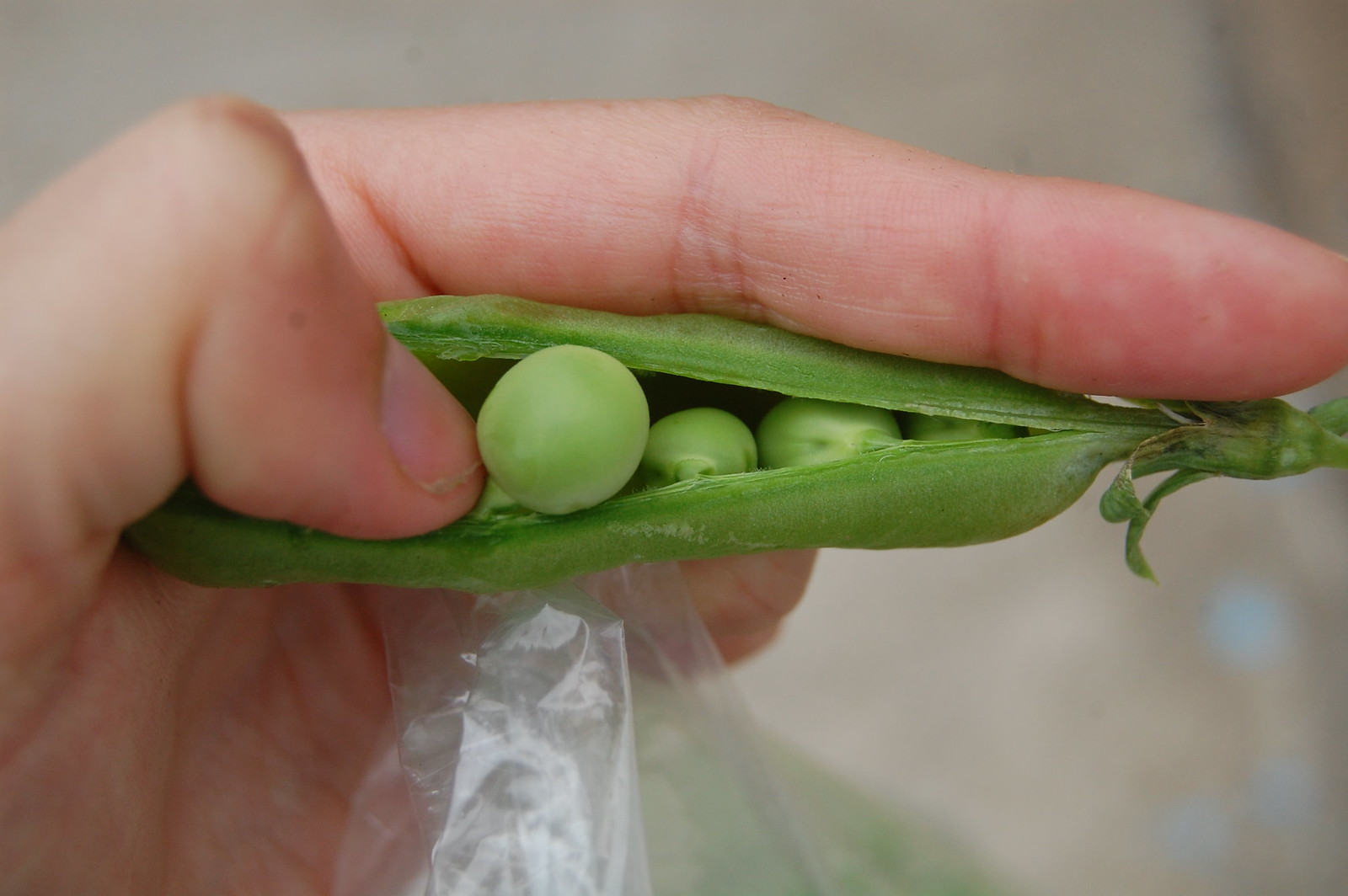This detailed close-up macro image captures a person holding a vibrant green pea pod in their left hand, which is split open to reveal lighter green peas inside. The person's thumb is pressing against one of the peas near the left side, causing it to partially pop out of the pod, while their index finger extends over the top towards the right. The pea pod, roughly the size of the person's palm to their index finger, is prominently displayed against a blurred gray background, making the colorful greens stand out. The hand also clutches a thin, translucent plastic bag beneath the pea pod, possibly containing more peas, although due to the bag being out of focus, the details are indistinct. At the tip of the pod, some leaves or other green material are visible, further adding to the naturalistic feel of the image.